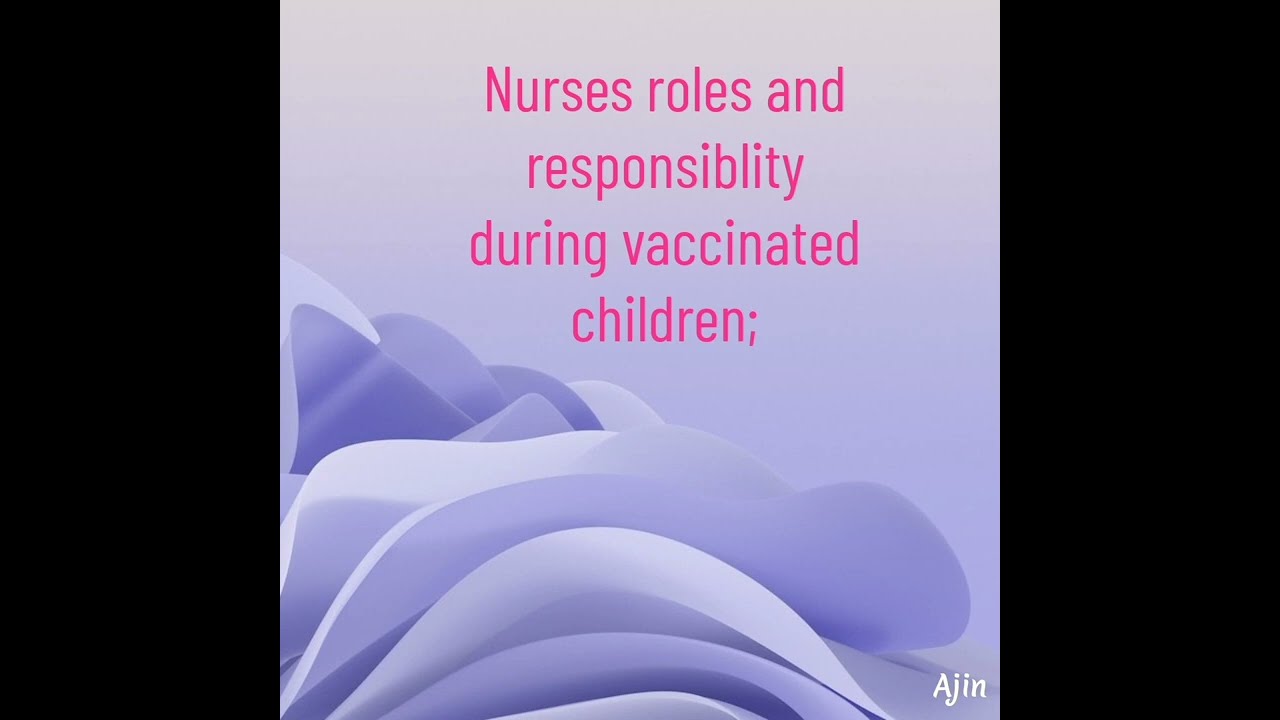The rectangular image features two vertical black bars on the left and right edges, each occupying about a fifth of the width. The central portion showcases a gradient background that transitions from white at the top to purple at the bottom, adorned with swirling, purplish cloud-like designs. An abstract, multi-layered graphic resembling petals or folded fabric in various shades of blue occupies the lower part of the central area. The main text, written in magenta or pink font, reads "Nurses' roles and responsibilities during vaccinating children." In the bottom right corner, the white text "AJIN" is visible.